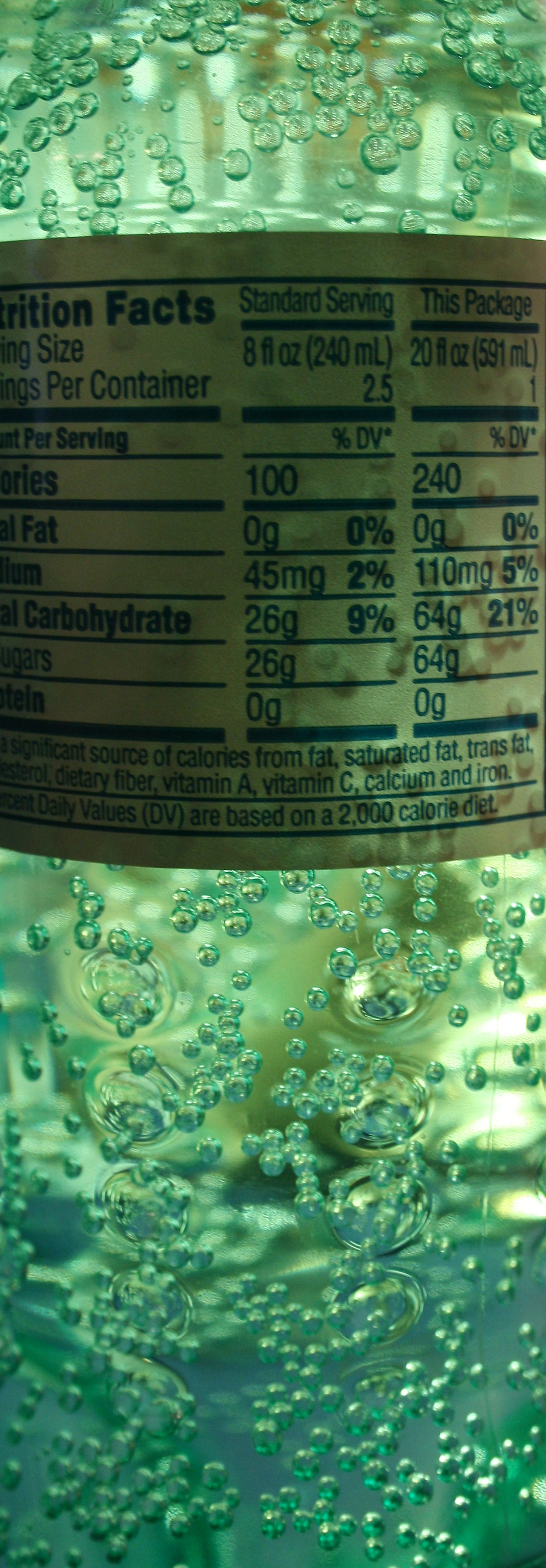The image showcases a close-up view of a green-tinted bottle, either made of plastic or glass, filled with a clear liquid. The liquid inside the bottle is effervescent, with numerous bubbles rising vertically from the bottom to the top, including both small circular bubbles and larger ones. The bottle is partially illuminated, giving it a brighter, almost glowing appearance. 

A partial nutritional facts label is visible on the upper half of the bottle, though it is partially obscured and difficult to read due to the lighting and angle. The label is white with black text and includes details such as "Nutrition Facts," "Standard Serving," and numerical values like "8 fluid ounces," "100," "0g," "45mg," "26g," and "0." Additional information about various vitamins and nutrients, including Vitamin A, Vitamin C, and Iron, can also be seen on the label.

The overall look and bubbles suggest that the bottle likely contains a carbonated beverage, possibly a clear soda like Sprite or Sierra Mist, although the exact type of liquid is uncertain.